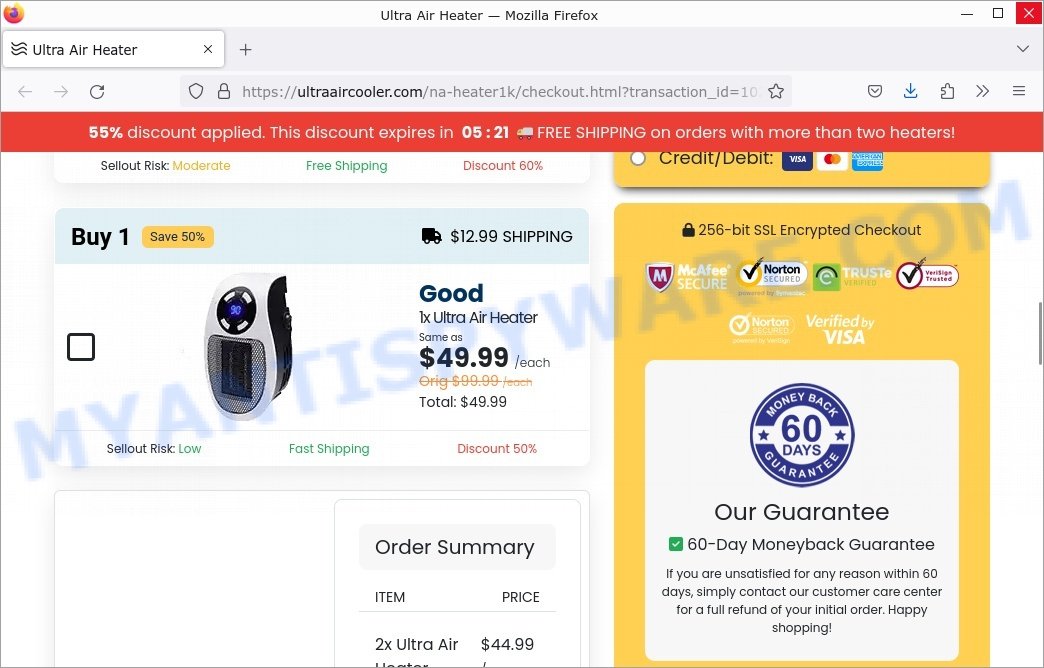The image depicts a promotional webpage for the Ultra Air Heater viewed in Mozilla Firefox. 

**Header Details:**
- Top-left: Mozilla Firefox icon.
- Top-center: "Ultra Air Heater" text.
- Top-right: Red "X" symbol for closing the window.

**Banner Section:**
- A tab label named "Ultra Air Heater."
- An address bar indicating the web page's URL.
- A prominent red banner stating, "55% discount applied," along with "This discount expires 5/21" and "Free shipping on orders with more than two heaters."

**Main Product Listing:**
- The listing is for a white and black Ultra Air Heater.
- Price prominently displayed: $90.
- Promotional text: "Buy One, Save 50%."
- Shipping cost: $12.99.
- Details of the deal: "Good, 1X Ultra Air Heater — $49.99 each," originally priced at $99.99 each.
- Total cost for one heater is listed as $49.99.
- Additional offers include: "Sell at risk, low," "Fast shipping," and "50% discount."

**Order Summary:**
- Itemized price for two Ultra Air Heaters: $44.99 each.
- Security features: "2256-bit SSL encrypted checkout," accompanied by icons for McAfee Secure and Norton.
- Money-back guarantee: "60-day guarantee" with a detailed paragraph explaining the terms of the guarantee.

This webpage effectively combines product details, promotional offers, and security assurances to motivate potential buyers.